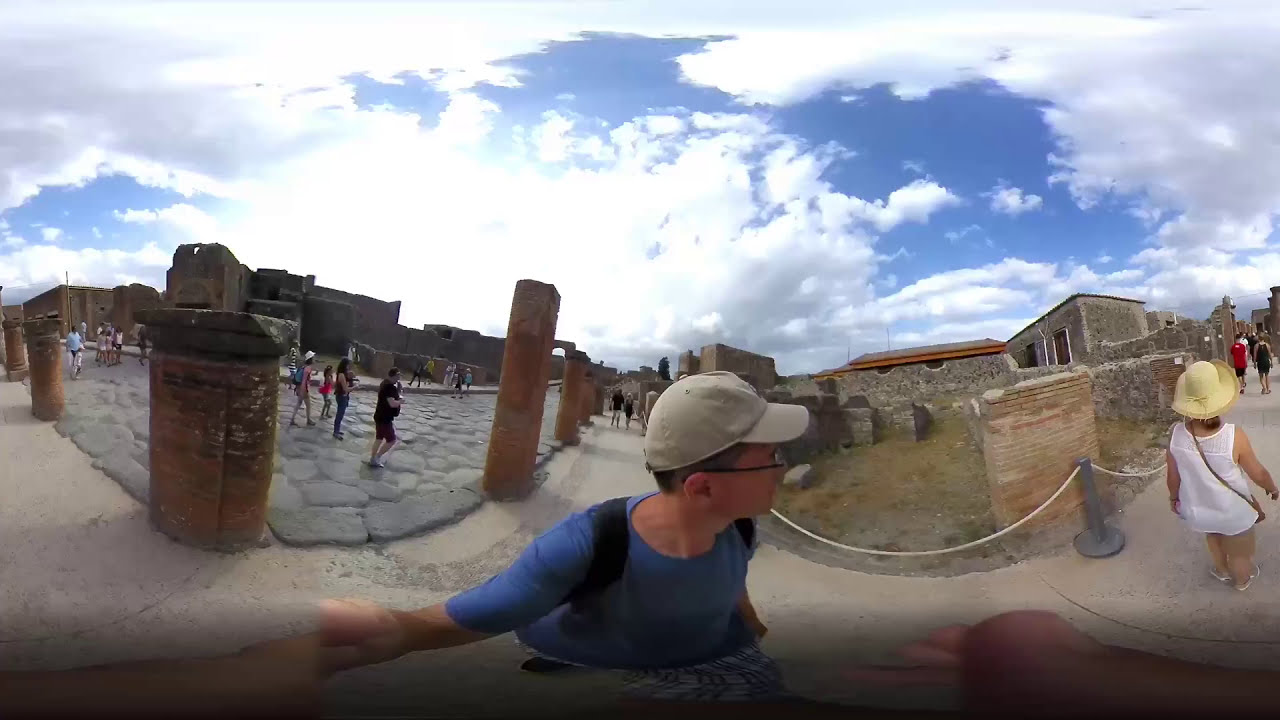In this fisheye lens photograph, a Caucasian man in the foreground, wearing a tan baseball cap, glasses, and a blue short-sleeved shirt with visible black backpack straps, looks to the right. He has short brown hair and dons plaid gray and white shorts with black shoes. Behind him, a woman in a white sleeveless top, a straw hat, and a brown sling bag draped over her right leg walks away down a pathway. She holds her hands in front of her as she moves forward.

The scene appears to be at a tourist site with ancient, adobe-like structures. The walkways are composed of cobblestone and various tiled rock formations glued together, forming intricate patterns. Tall, brown columns frame these paths, creating distinct walkways from left to right and towards the center.

Scattered about are tourists dressed in casual, sun-blocking attire such as hats and tank tops. The background features a sky dominated by gray and white clouds with hints of blue, with a bright white light on the left side where the sun breaks through. Numerous people can be seen in the distance, as the pathway extends towards groups of indistinct figures under the expansive, cloud-spotted sky. The fisheye effect distorts the image, giving it a warped, almost surreal quality.